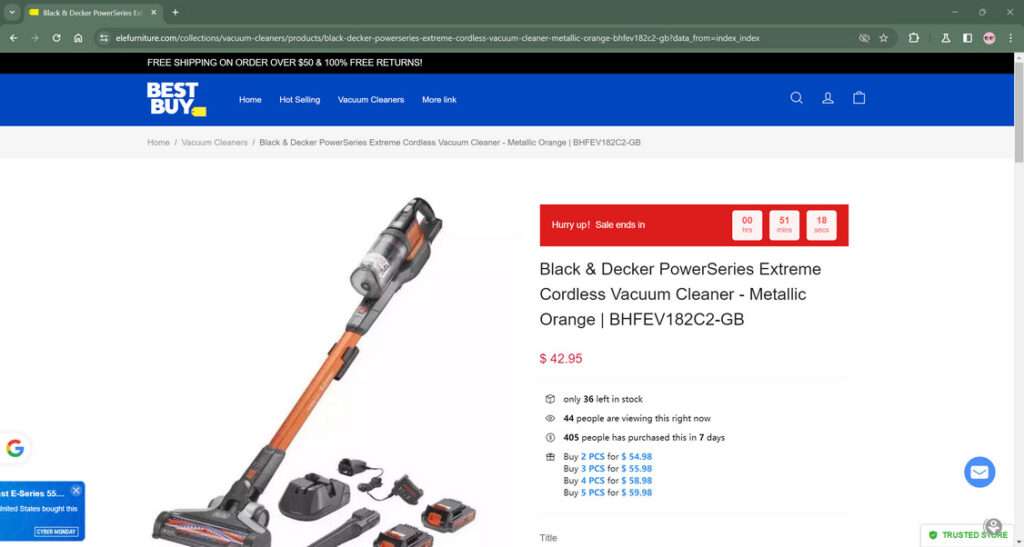This screenshot captures a section of the BestBuy.com homepage. At the very top, a black bar with white text announces, "Free shipping on orders over $50 and 100% free returns." Directly beneath this, a blue navigation bar features the Best Buy logo in the left corner, followed by links labeled "Home," "Hot Selling," "Vacuum Cleaners," and "More," accompanied by a search bar, a user account icon, and a shopping bag icon on the right.

Further down, additional navigation links read "Home," "Vacuum Cleaners," and "Black and Decker," leading to a specific product page for the "Power Series Extreme Cordless Vacuum Cleaner in Metallic Orange." The product's serial number is also listed.

A prominent red banner across the page urges, "Hurry Up! The Sale Ends In," with a countdown timer showing 51 minutes and 18 seconds remaining. This section includes details such as the product name—Black and Decker Power Series Extreme Cordless Vacuum Cleaner in Metallic Orange, the serial number, and the remaining stock, noting, "Only 36 left in stock." Additionally, real-time information indicates that 44 people are currently viewing the item and 405 have purchased it in the last seven days.

On the left side of the screenshot, there is an image of the vacuum cleaner itself, providing a visual reference for the featured product.